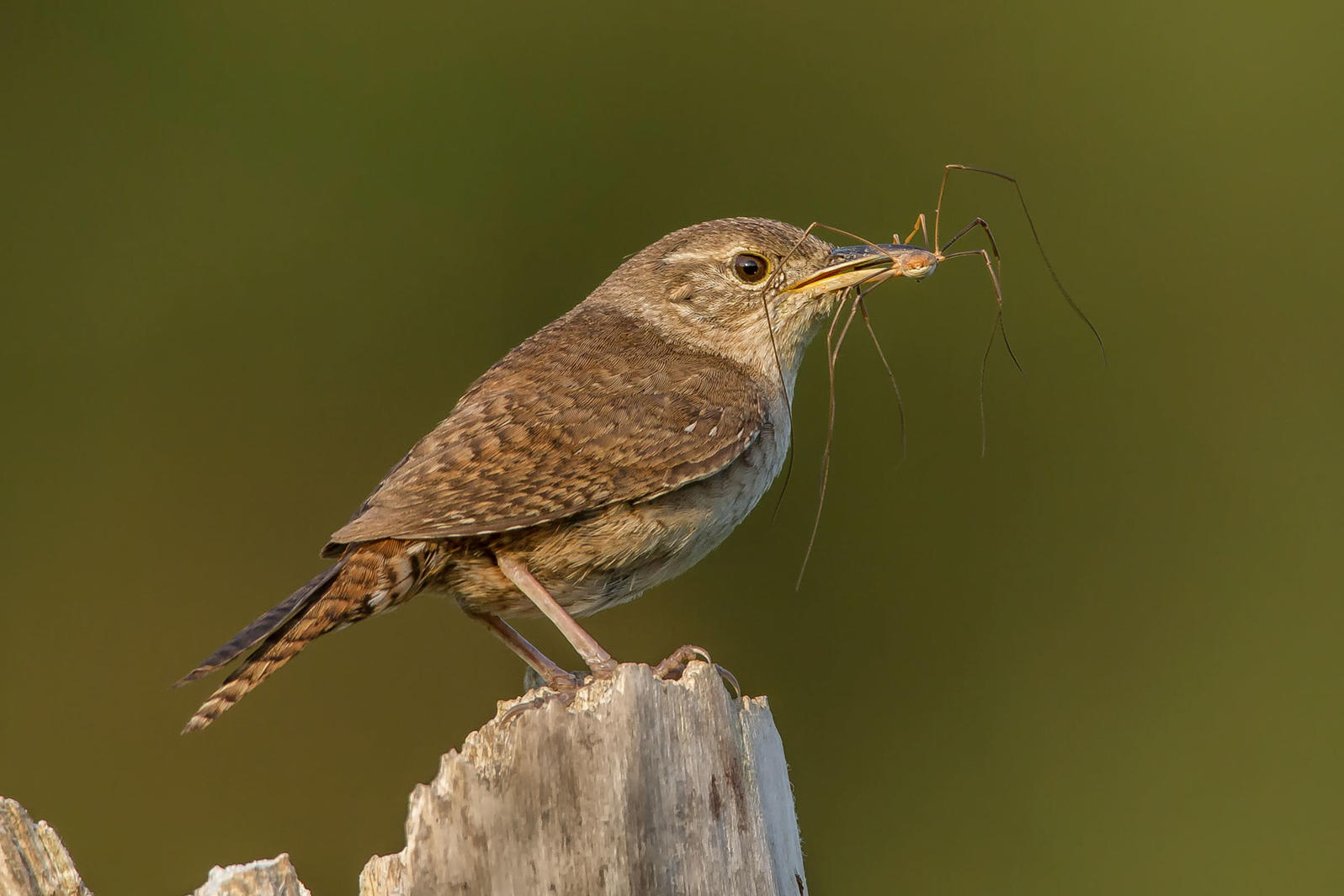The photograph captures a small brown bird, possibly a type of swallow or hummingbird, with dark eyes and thin brown legs. The bird is perched on a splintered wooden stump and is holding an insect, likely a daddy long-legs spider or large mosquito, in its beak. You can distinctly see the spindly legs of the insect sticking out. The bird features a dark pattern among its brown feathers, with subtle white dots under its tail and stripes of brown and gray. The background of the image is a blurred olive green, suggesting foliage, and the lighting indicates that the sun is either rising or setting, casting a soft natural light over the scene. The composition places the bird slightly off-center to the left, with more of the stump visible at the bottom left corner. The overall colors in the photograph are primarily brown and green, with hints of white and orange.